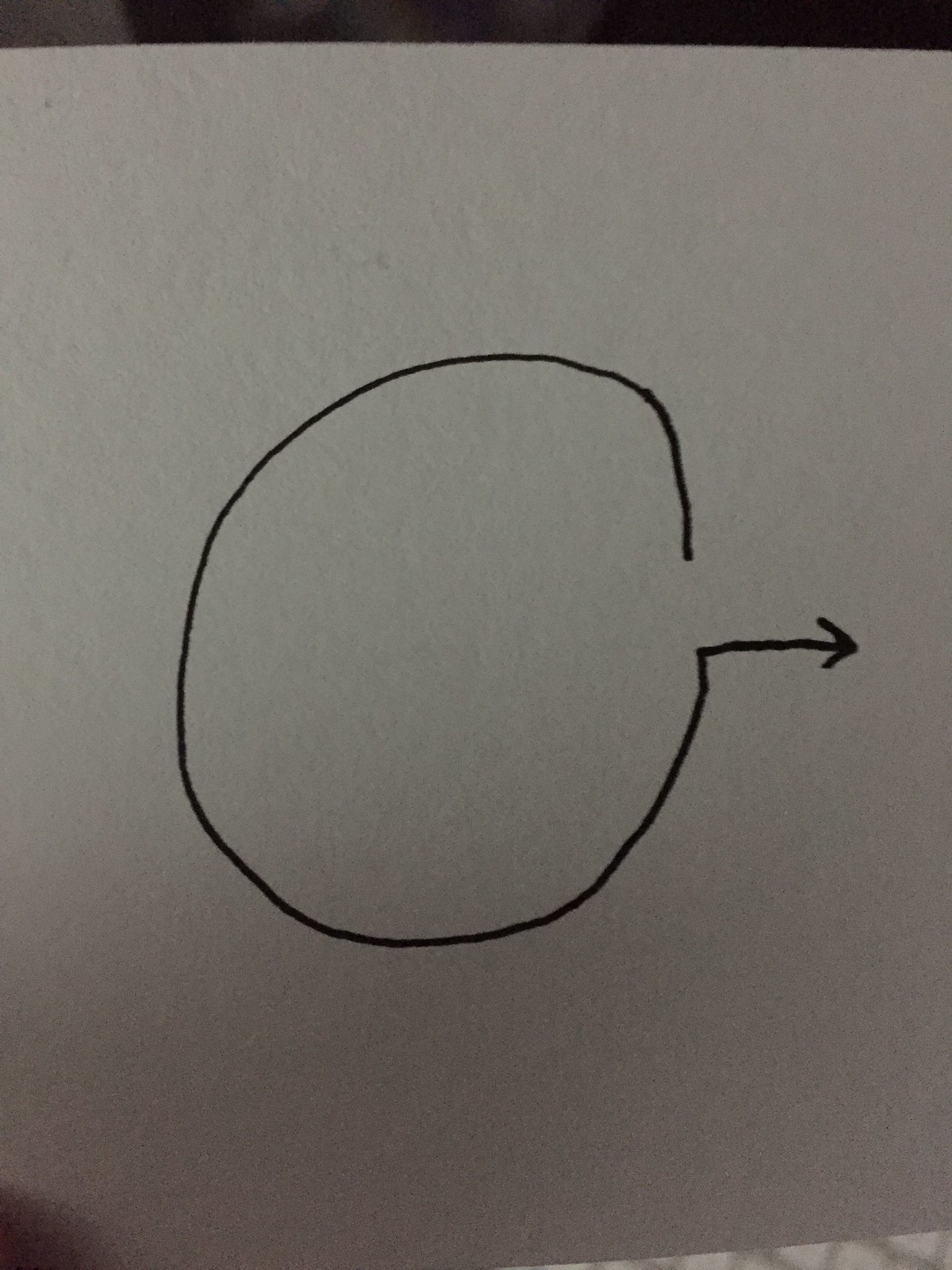The image displays a hand-drawn figure on a plain white sheet of paper positioned centrally within the frame. The drawing, executed with a pen, features an almost-complete circle that diverges into an arrow pointing rightward from the lower part of the circle. The circle has a slight protrusion near the upper-right side and appears somewhat flattened on the lower-left side, with evident indications of areas that have been retraced. In the very bottom left corner of the image, a small shadow is visible, and along the bottom edge in the lower right corner, there is a noticeable shadow extending beyond the paper onto a dark background. The background around the paper is very dark, adding contrast and highlighting the simple yet striking focus of the pen-drawn circle and arrow.